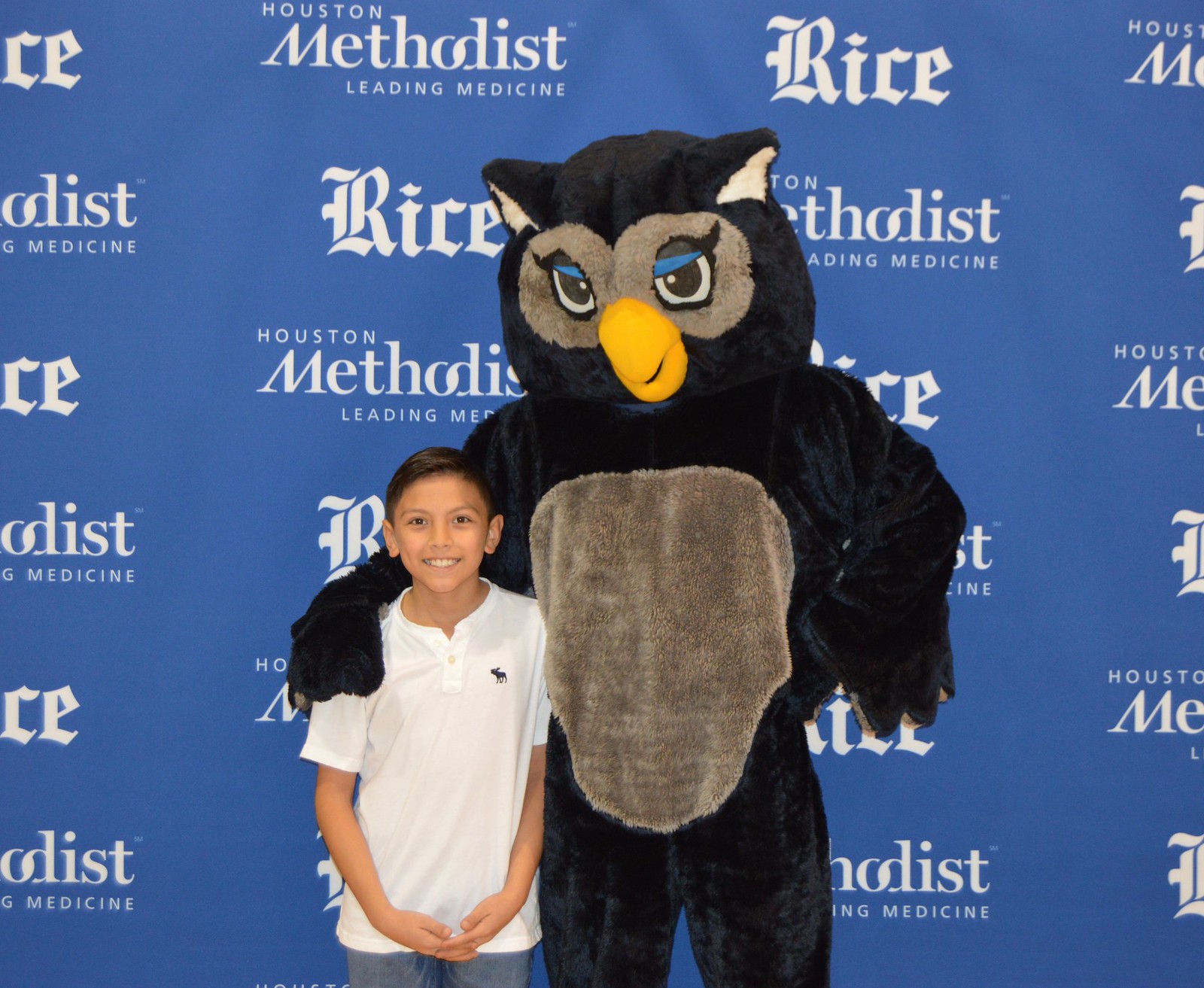In the photograph, a young boy with short brown hair is posing with a large owl mascot against a blue backdrop adorned with the repeating white text, "Rice" and "Houston Methodist Leading Medicine." The boy, who is wearing blue jeans and a white t-shirt featuring a moose logo, stands on the left with his hands clasped at his waist and a smile on his face. The mascot, likely representing the Rice Owls, is predominantly blue with a brown belly and face, white ears, and a bright yellow beak. The owl has gray wings and gray around its eyes, accentuated with blue eyeshadow and black eyeliner. The mascot's right wing is draped over the boy’s right shoulder, completing the friendly pose.